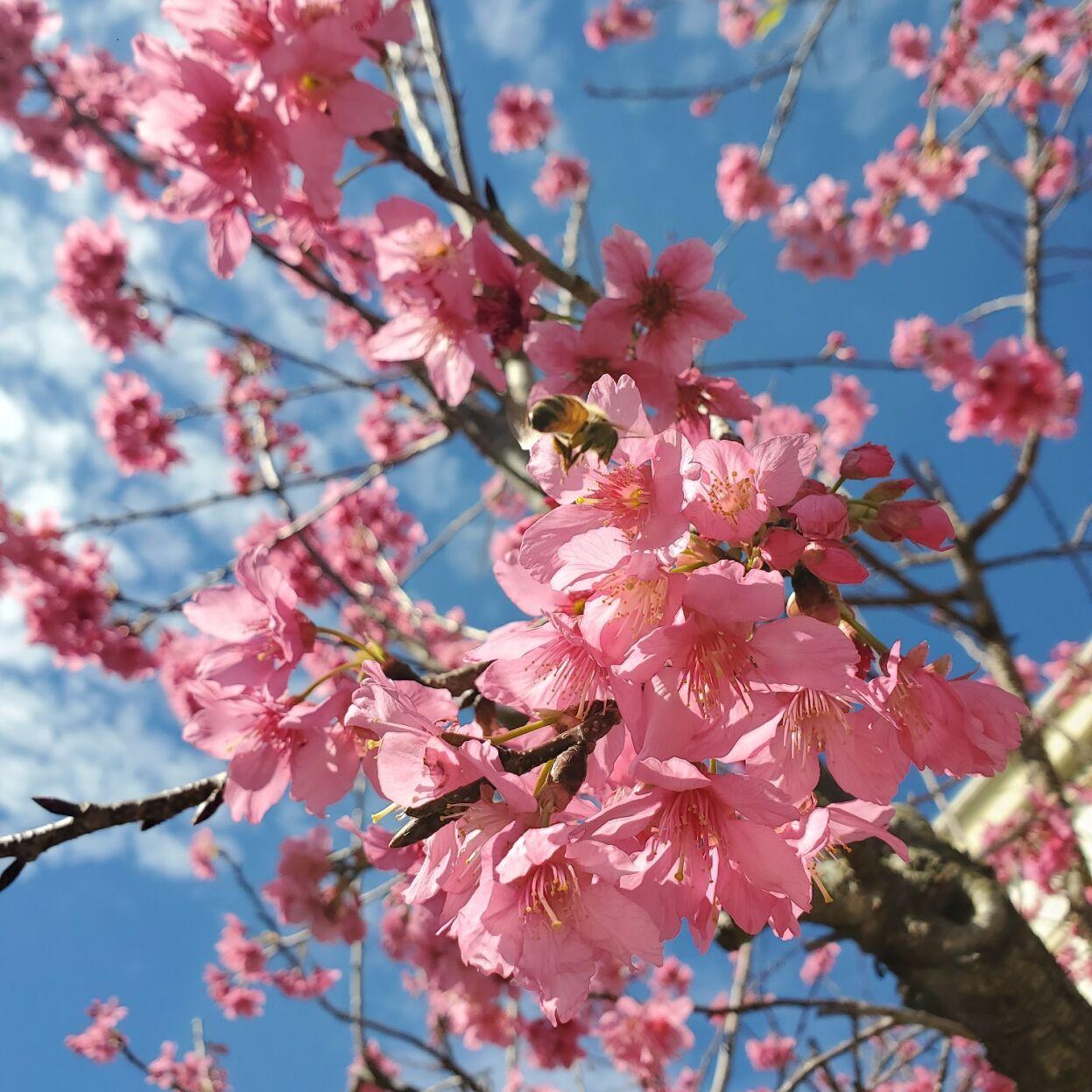This vibrant close-up color photograph captures the essence of spring with its detailed portrayal of cherry blossoms set against a vivid blue sky with scattered white cirrus clouds. The focus is on a cluster of light pink cherry blossoms, which showcase darker pinkish-orange stamens at their centers. A bee, characterized by its yellow and dark orange striped body with black ends and head, is seen in mid-flight toward one of the blossoms, likely in the act of pollination. The bee's wings are a blur, suggesting their rapid movement. The dark brown branches of the cherry blossom tree stretch skyward, with some extending high up into the frame. In the lower right, there is a glimpse of what appears to be a cream-colored cornice of a building, hinting at the photograph being taken in an outdoor, possibly urban, setting. The photograph's composition highlights the delicate beauty of the cherry blossoms while subtly incorporating elements of the surrounding environment.